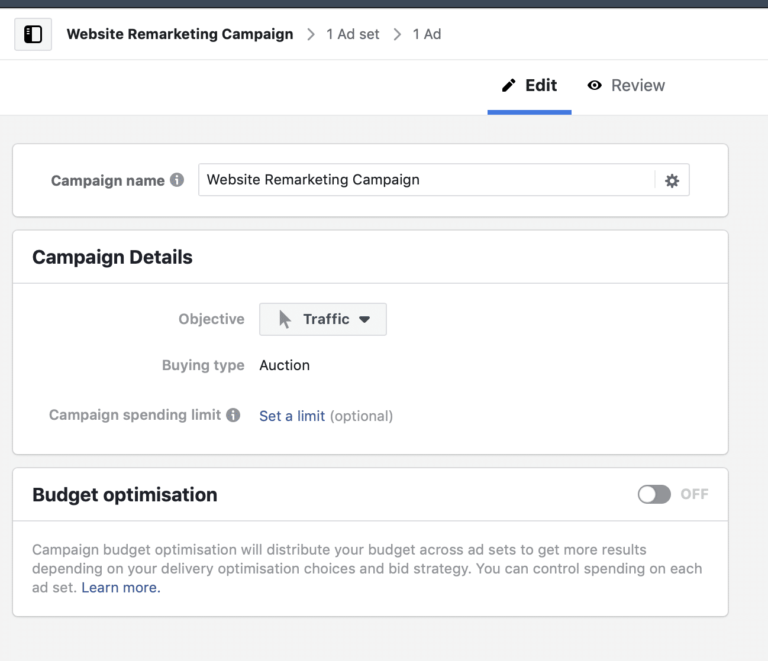This is a detailed screenshot from a Website Remarketing Campaign interface. On the right side of the interface, there are two buttons: an "Edit" button and a "Review" button, with the "Edit" button prominently underlined.

The "Edit" page is divided into three distinct sections, each set against a clean white background. 

1. **Campaign Name Section**:
    - This section is enclosed in a white rectangular box.
    - It is labeled "Campaign Name".
    - There is a small white text bar displaying the name "Website Remarketing Campaign".

2. **Campaign Details Section**:
    - This section is also enclosed in a white rectangular box.
    - The title "Campaign Details" heads this section.
    - Under "Campaign Details", there are three settings:
        1. **Objective**:
            - This setting includes a drop-down box currently set to "Traffic".
        2. **Buying Type**:
            - Labeled directly as "Auction".
        3. **Campaign Spending Limit**:
            - A prompt labeled "Set a limit (optional)".

3. **Budget Optimization Section**:
    - This final section is in a white rectangular box.
    - The title "Budget Optimization" is at the top.
    - This feature is toggled off.
    - There is an informative line stating: "Campaign budget optimization will distribute your budget across ad sets to get more results depending on your delivery optimization choices and bid strategy. You can control spending on each ad set. Learn more."

The overall layout is user-friendly, with clear divisions to easily locate and adjust the various aspects of the campaign.